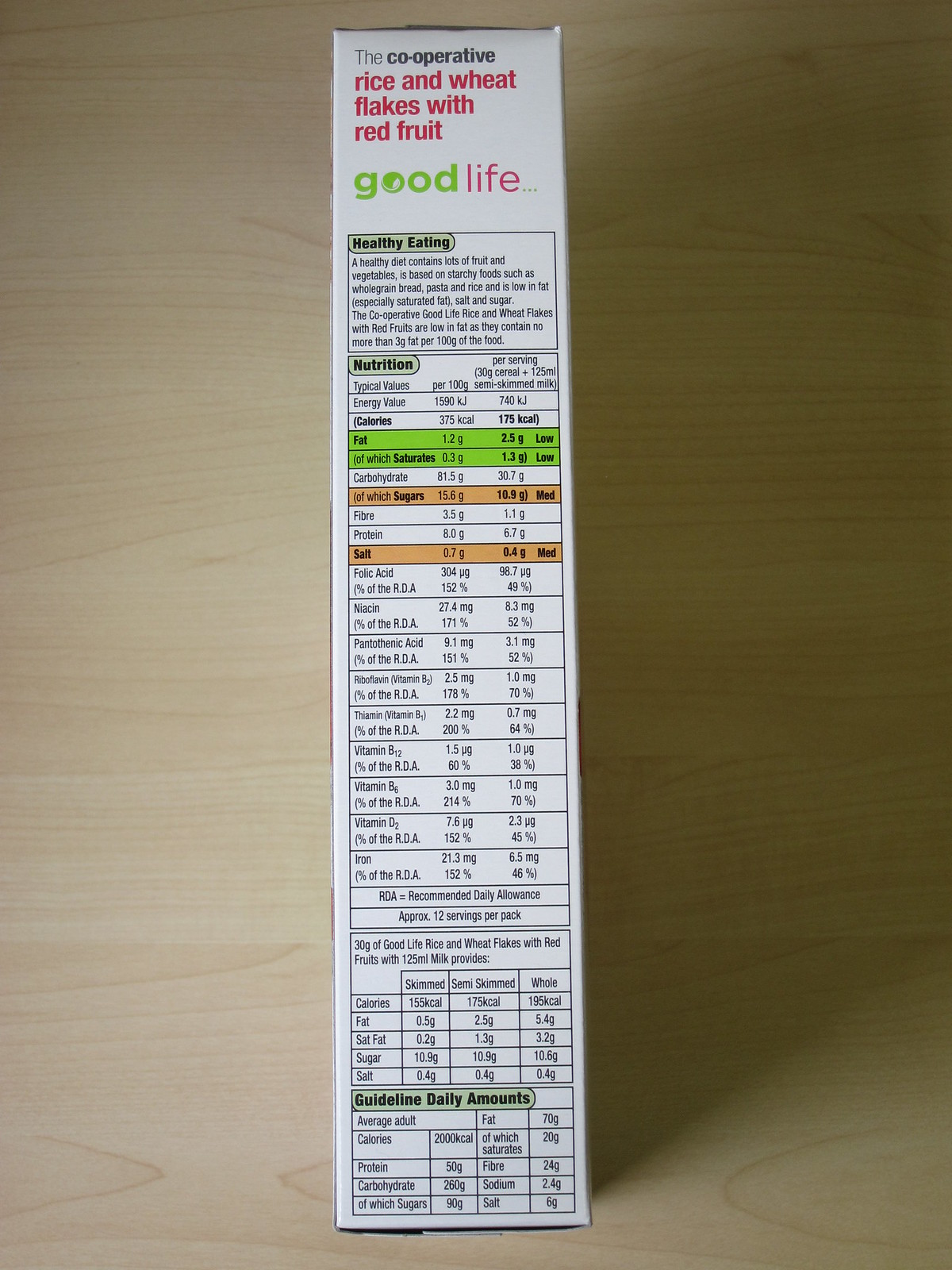A white product box, turned on its side to reveal intricate details, rests upon a light brown wooden surface. The refined wood grain patterns add a touch of natural elegance to the setting. Captured from a top-down perspective, the visible side of the box prominently displays the brand's information. At the top, bold text in black, red, and green announces "Cooperative Rice and Wheat Flakes with Red Fruit." Directly underneath, the tagline "Good Life" is printed. The rest of the box side is populated with comprehensive details about the product, including sections on healthy eating, nutritional information, and guideline daily amounts. These sections feature well-organized tables that provide consumers with essential dietary information. The meticulous layout contributes to a clear and informative presentation.